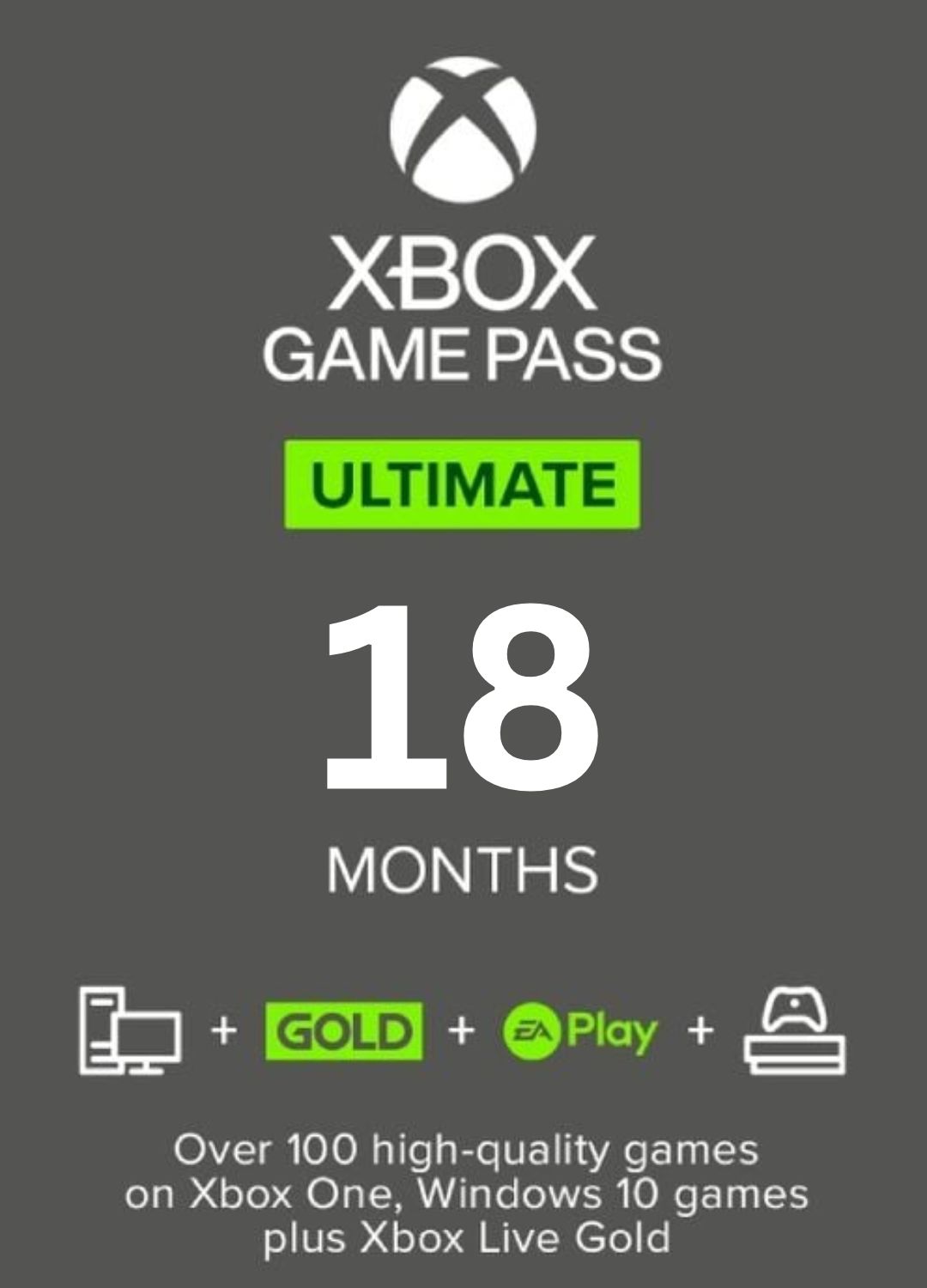The image features a promotional card for the Xbox Game Pass Ultimate, displayed in portrait mode. The background is a dark gray, giving the card a sleek and premium appearance. Positioned prominently in the upper center is the iconic Xbox logo, set within a white circle and featuring the signature green "X." Directly beneath this, in bold white text, the card announces "Xbox Game Pass."

Further down, there's a green rectangular button with the word "Ultimate" boldly written in white, signifying the tier of the service being promoted. Just below this button, "18 months" is displayed in white font, indicating the duration of the subscription.

The card also features several icons and text descriptions to highlight the benefits included in the Ultimate package: devices compatibility, Xbox Live Gold, and EA Play, showcasing a comprehensive gaming experience across multiple platforms. Additionally, it boasts access to over 100 high-quality games on both Xbox One and Windows 10.

The overall design maintains a consistent color palette of dark gray, light green, and white, providing a clean and visually engaging presentation. This card serves as an advertisement for the Xbox Game Pass Ultimate, emphasizing an 18-month subscription period.